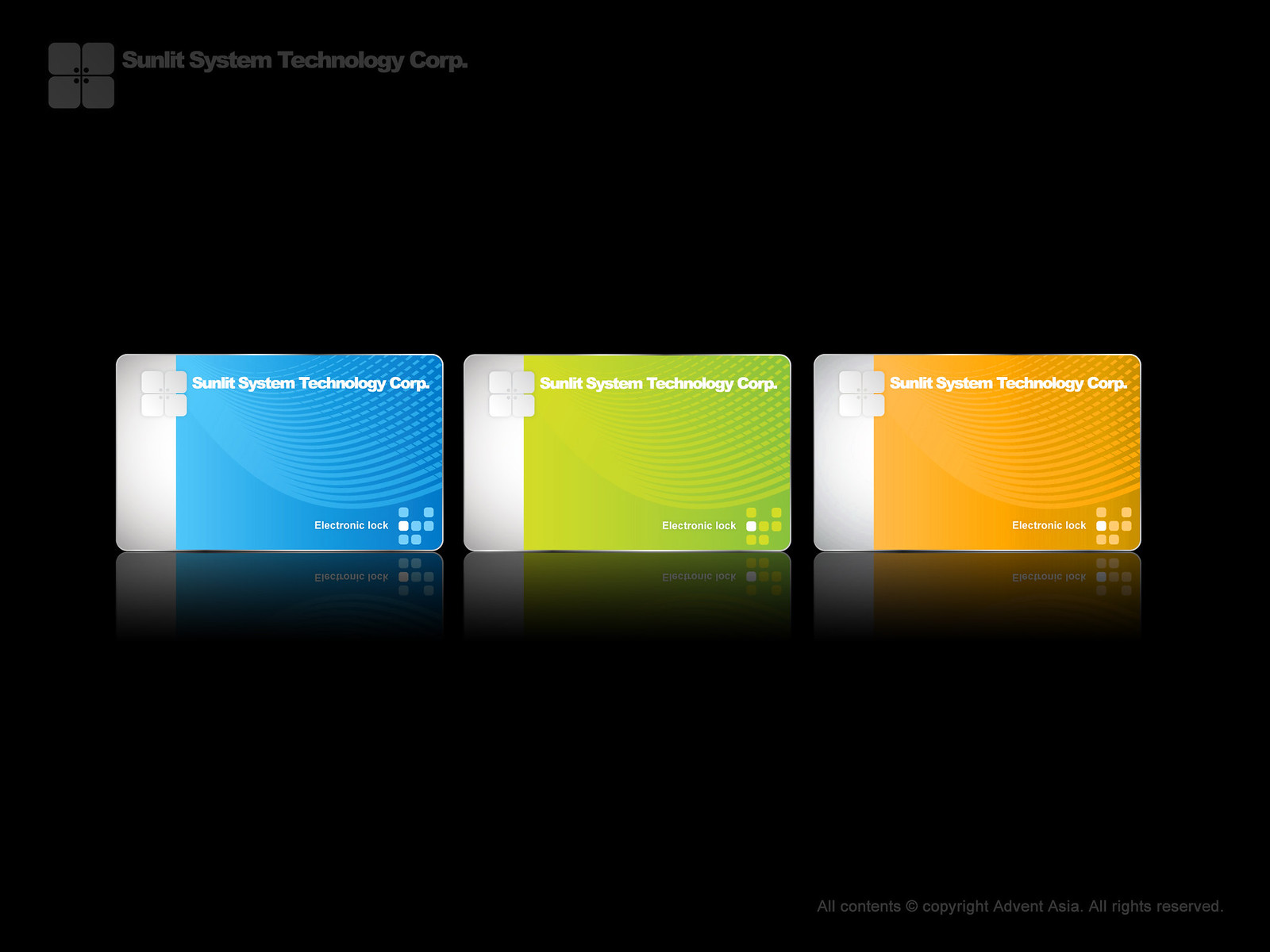The image features a solid black background, with three electronic key cards prominently placed in the center in a horizontal alignment. Each card is the size of a driver's license or a credit card and shares a similar design layout. On the left edge of each card is a distinctive silver strip, with the main body of the cards showcasing bright colors: the left card is blue with wave-like patterns, the middle card is lime green, and the right card is tangerine orange. At the top of each card is the text "Sunlit System Technology Corp." accompanied by a logo resembling a flower made up of four squares. In the bottom right corner of each card, the words "Electronic Lock" are displayed. Additionally, the left card features a unique arrangement of small squares near the "Electronic Lock" text, forming a line of three squares with one lit in white, two squares on top, and two below. In the top left corner of the entire image, the text "Sunlit System Technology Corp." is printed in a very light gray font, along with the same flower-like logo. The image has no people, animals, plants, or trees. At the bottom right corner of the photograph, there is a disclaimer: "All contents copyright Advent Asia, all rights reserved."